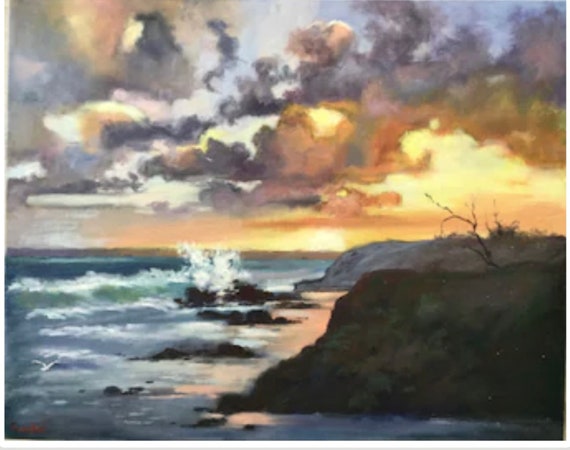This artwork, possibly an oil or watercolor painting, depicts a stark and evocative stormy coastline, likely reminiscent of the rugged Pacific coast. The ocean, characterized by deep grays, dark blues, and white foam, crashes energetically against shadowed, rocky outcrops on the shore. In the foreground, the rocky dunes are sporadically dotted with sparse, unhealthy foliage, mostly bare sticks, while a faint strip of sand catches the sun's reflection. Above, the sky is a dramatic tapestry of colors, transitioning from muted dark gray clouds to the warm hues of sunset or sunrise, featuring gold, yellow, orange, rose, light pinks, and blues. Despite the stormy setting, the sun peeks through the clouds, adding a touch of warmth to the turbulent scene. The painting's abstract nature and rich, varied palette create a sense of both beauty and intensity in the depicted natural chaos.